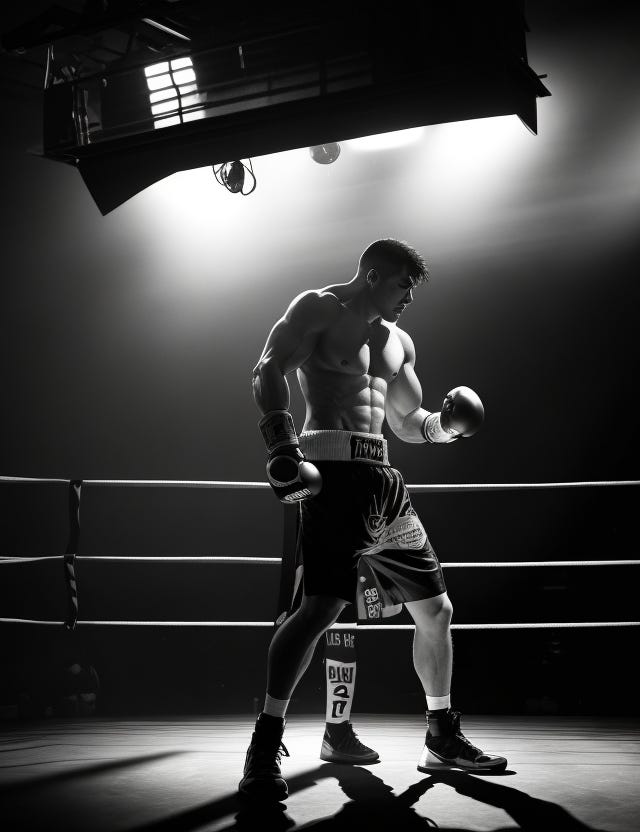The photograph captures a striking black and white image of a muscular boxer standing in the ring, adorned in proper boxing attire including gloves, trunks with a misaligned text, a belt, and sneakers. The boxer, with very short hair and jagged muscle definition, stands facing off to his left, gazing out towards the right side of the image. The dimly lit background is predominantly dark with spotlights casting dramatic highlights and shadows, contributing to the enigmatic atmosphere of the scene. Intriguingly, between the boxer’s legs, there is an unexplained third leg on the floor, with the ring ropes overlapping it, making the anomaly conspicuous and puzzling. This third leg, lacking a visible source, adds an odd, almost surreal element to the photograph, as if hinting at a deliberate manipulation or digital artifact within this professionally taken image.